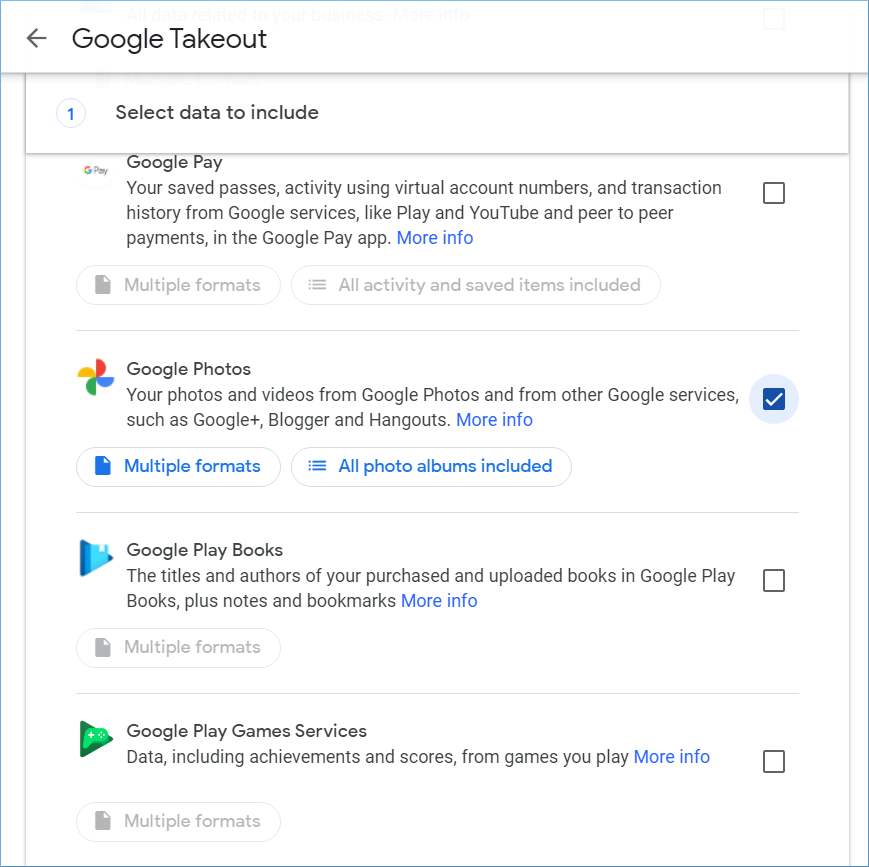The image features a Google Checkout interface, prominently displaying a header with the text "Google Checkout" at the very top left corner, written in black. Below the header is a bar with the label "Select Data to Include" also written in black. Multiple fields are listed vertically under this section, each representing different Google services. These fields include Google Pay, Google Photos, Google Play Books, and Google Play Games Services. 

In the checklist, Google Photos is the only service that is checked. Underneath Google Photos, there is a description stating "Your photos and videos from Google Photos and from other Google services such as Google Plus, Blogger, and Hangouts." Additionally, there is a link labeled "More info," written in blue, and next to it, an icon with the text "Multiple formats." Below this, another icon is present, stating "All Photo Albums included."